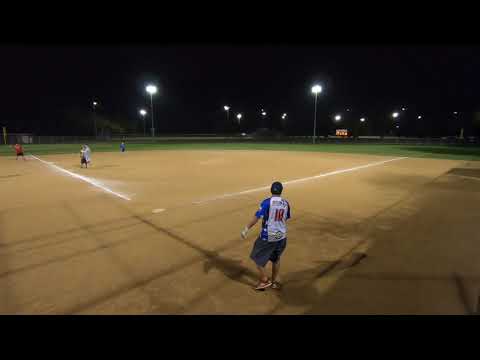This nighttime photograph captures an expansive view of a baseball field from the perspective of home plate, looking outward. The field, bathed in the glow of several tall floodlights, features distinct white lines and a visible home plate. Atmospheric shadows hint at grandstands or surrounding structures beyond the frame's edges. The brown, slightly orange-colored sand of the infield occupies the bottom half, curving gracefully at the center.

Prominently, a man stands slightly right of center, his back turned to the camera. He is dressed in a white and blue jersey adorned with red numbers, blue jean shorts, and sneakers. He sports a black cap, adding to his athletic appearance. His tan skin glows under the field's lights, and the jersey may bear the number 15. Scattered around the field are other players: one in a red shirt, another in white, and a third in blue, positioned closer to the outfield. The lush green grass of the outfield stretches toward a distant scoreboard, barely discernible against the black sky. Thick black strips at the top and bottom of the image frame the scene, focusing the viewer's attention on the vibrant life of this night-time baseball game.